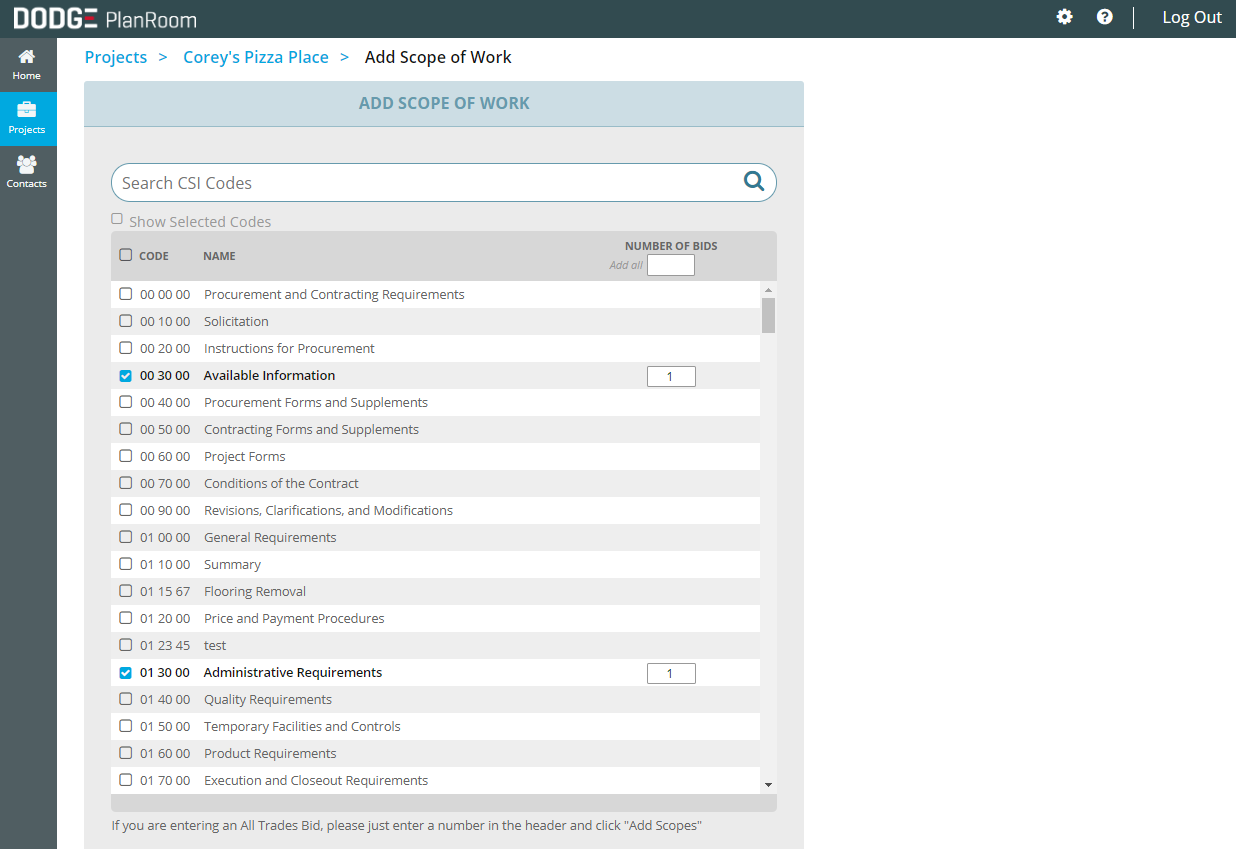The image showcases a user interface of a program identified in the top left-hand corner as "Dodge Plan Room." On the left side of the screen, a taskbar is visible featuring options labeled "Home," "Projects," and "Contacts." The "Projects" tab is highlighted in blue, indicating the active section.

In the main viewing area, a navigation flow is displayed, starting with "Projects" and progressing through an arrow to "Corey's Pizza Place," followed by another arrow to the current section, "Add Scope of Work." Below this flow, there is a search text box labeled "Search CSI Codes" for finding specific construction codes.

A detailed table occupies the central part of the screen, organized with headers titled "Code," "Name," and "Number of Bids." Each entry in the table lists the CSI code and its corresponding name, with two entries also displaying the number of bids. In this particular view, two codes are marked with blue checkmarks: code "003000," named "Available Information," and code "013000," named "Administrative Requirements."